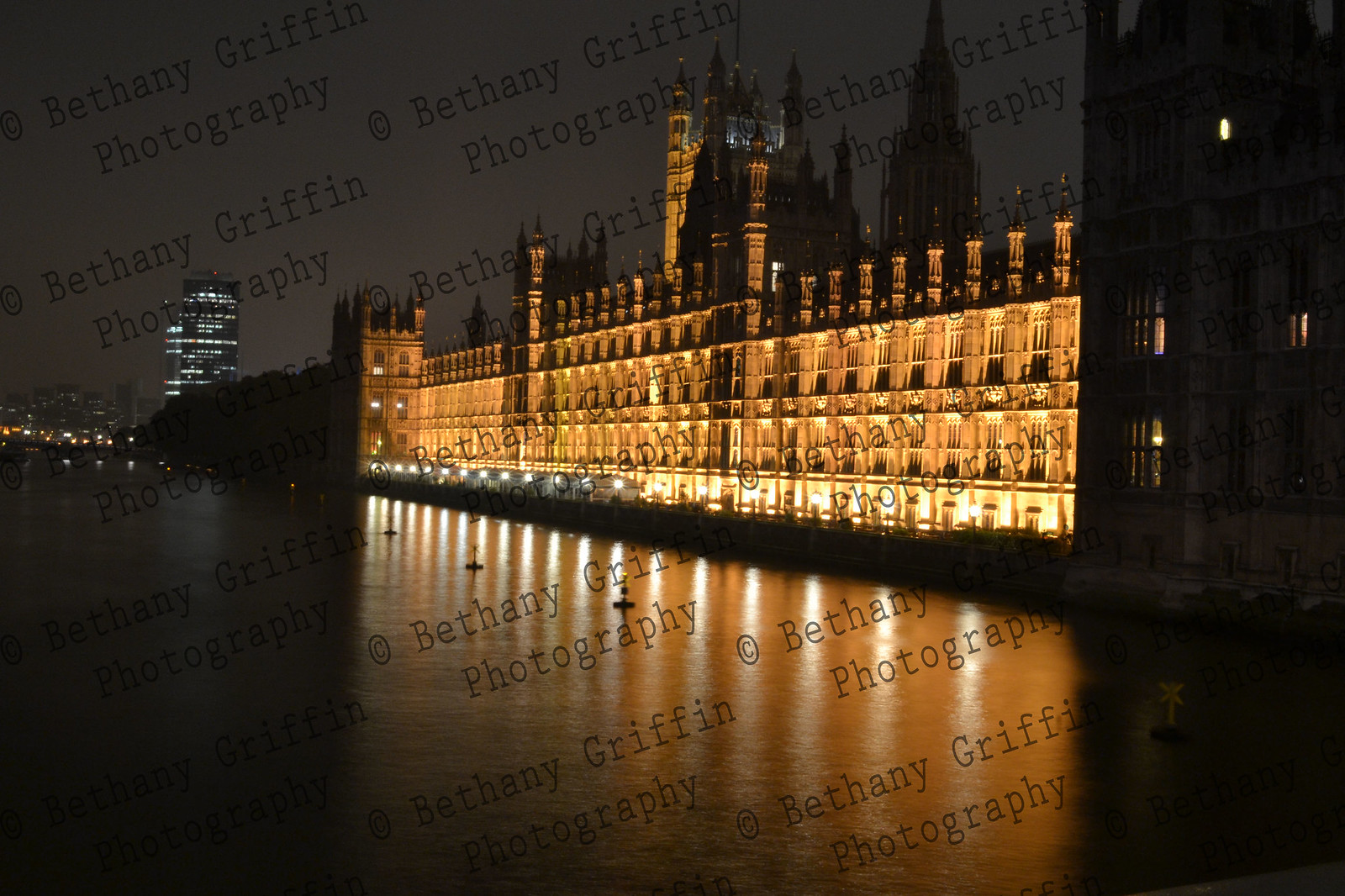This nighttime photograph, attributed to Bethany Griffin Photography, captures a grand, illuminated building that strongly resembles a castle or parliament-style structure, possibly the British Parliament on the Thames River. The building is set against a backdrop of water with its lights beautifully reflecting off the calm surface. The scene hints at an overcast sky with some light subtly illuminating the clouds. In the background, there are numerous tall skyscrapers with their lights on, indicating a bustling city. The photograph features a copyright watermark by Bethany Griffin Photography, placed multiple times and at an angle, adding a layer of authenticity. The dark tones dominate the image, especially on the sides, accentuating the brilliantly lit architecture and enhancing the serene yet majestic night-time scene.